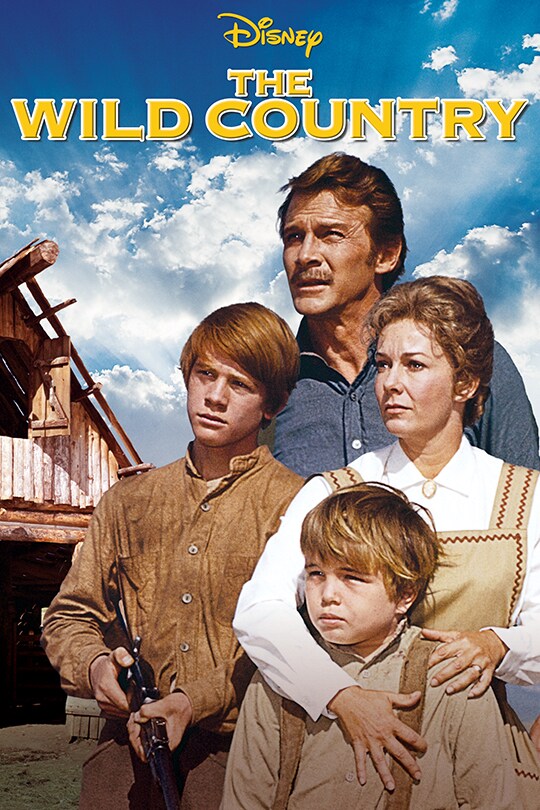This is a detailed poster for the Disney movie "The Wild Country," which has the appearance of a VHS tape cover. The image features a rugged-looking man with a sun-beaten face, blue shirt, and reddish hair standing behind his family. His wife, donned in an apron-style dark dress over a long-sleeve white shirt with her hair pinned up, stands protectively with her arm draped around their younger son. This smaller boy, who looks about seven years old, has a chubby face and wears brown suspendered pants over a tan shirt. Beside the mother is their older son, a boy with short, combed-over red hair, holding a shotgun or rifle and looking with a resolved expression towards something off-frame, indicating readiness to defend. The family of four - a father, mother, and two sons - stands in front of an old wooden barn under a strikingly bright Disney-blue sky with some clouds. Above the family's heads, the title "The Wild Country" is displayed in large letters, with the word "Disney" in smaller yellow print above it. All family members direct their gaze towards the left front side of the poster, hinting at an unseen tension.